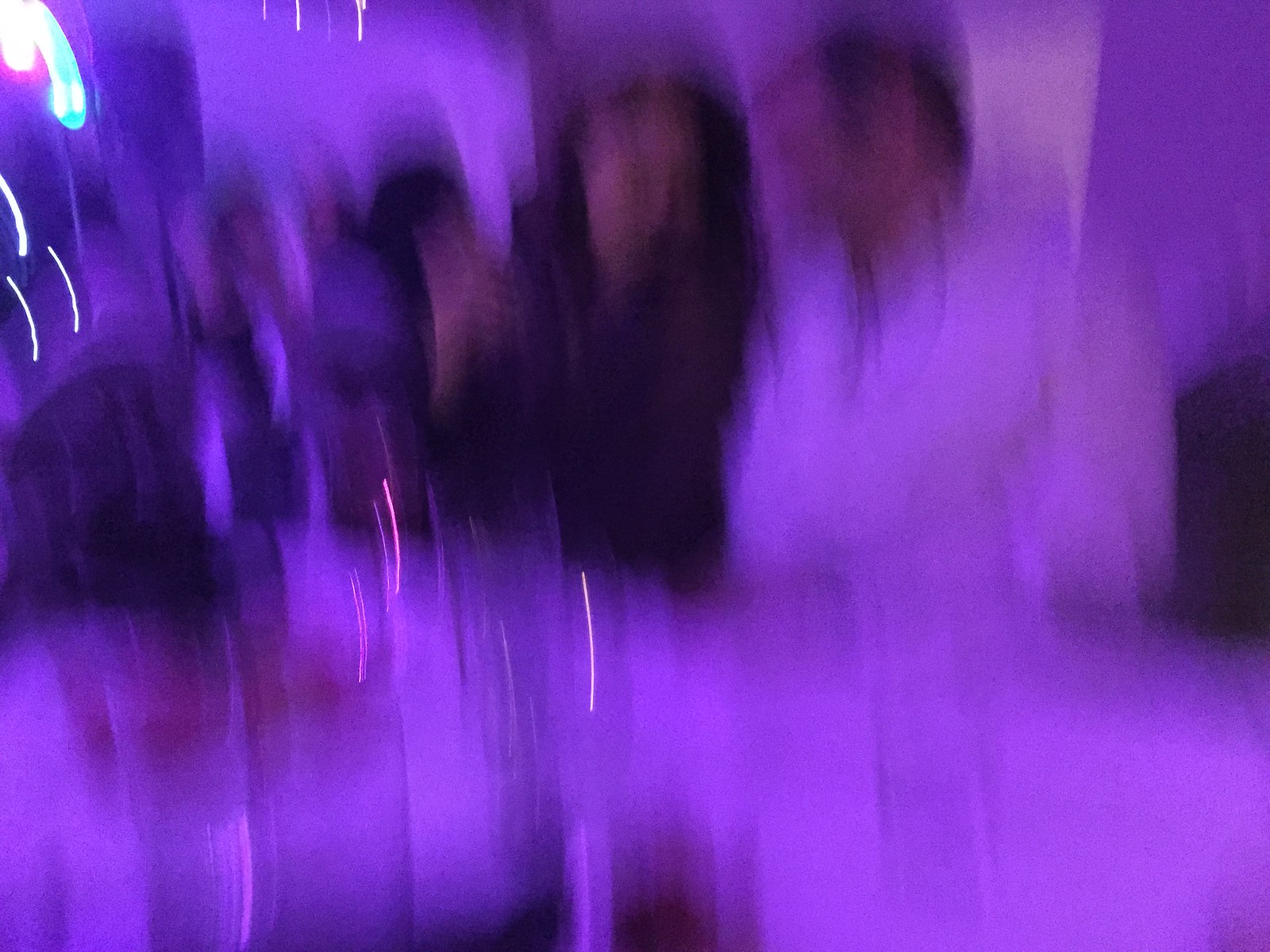This is an extremely blurry photograph immersed in a pervasive purple glow, suggesting it was taken in a uniquely lit indoor environment, such as a bar, bowling alley, or roller skating rink. At the center of the image, two human figures are discernible, seated at what appears to be a bright purple or possibly white table that reflects the surrounding lights. The man, with short dark or potentially gray hair, is dressed in a light-colored long-sleeved shirt and is engaged in conversation with a woman to his left. The woman has long, straight dark hair left loose and is wearing a dark-colored top or dress. Her hand is raised, possibly holding a glass or gesturing while she speaks. In the distractingly blurry background, additional people can be faintly seen socializing near neon lights positioned in the upper left corner. Several clear glasses are placed on the table, catching reflections from the ambient lighting. This image seems to capture a lively, albeit indistinct, social setting.